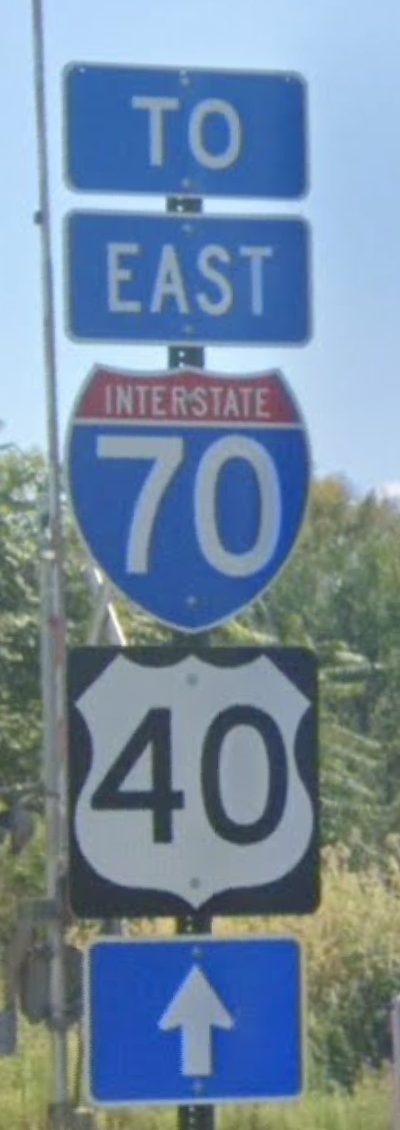This photograph features a series of five road signs stacked vertically on a single pole, set against a clear blue sky with a backdrop of green trees and bushes. The topmost sign is a blue rectangle with "TO" in white letters. Directly below it is another blue rectangle with "EAST" also in white letters. The third sign is an interstate shield, with the top portion in red and the word "INTERSTATE" in white font, followed by a blue section with the number "70" in white. Below this is a black square sign that features a white shield shape with the number "40" in black. The bottom sign is a blue rectangle with a white arrow pointing upward. All the signs are mounted on a singular black pole.